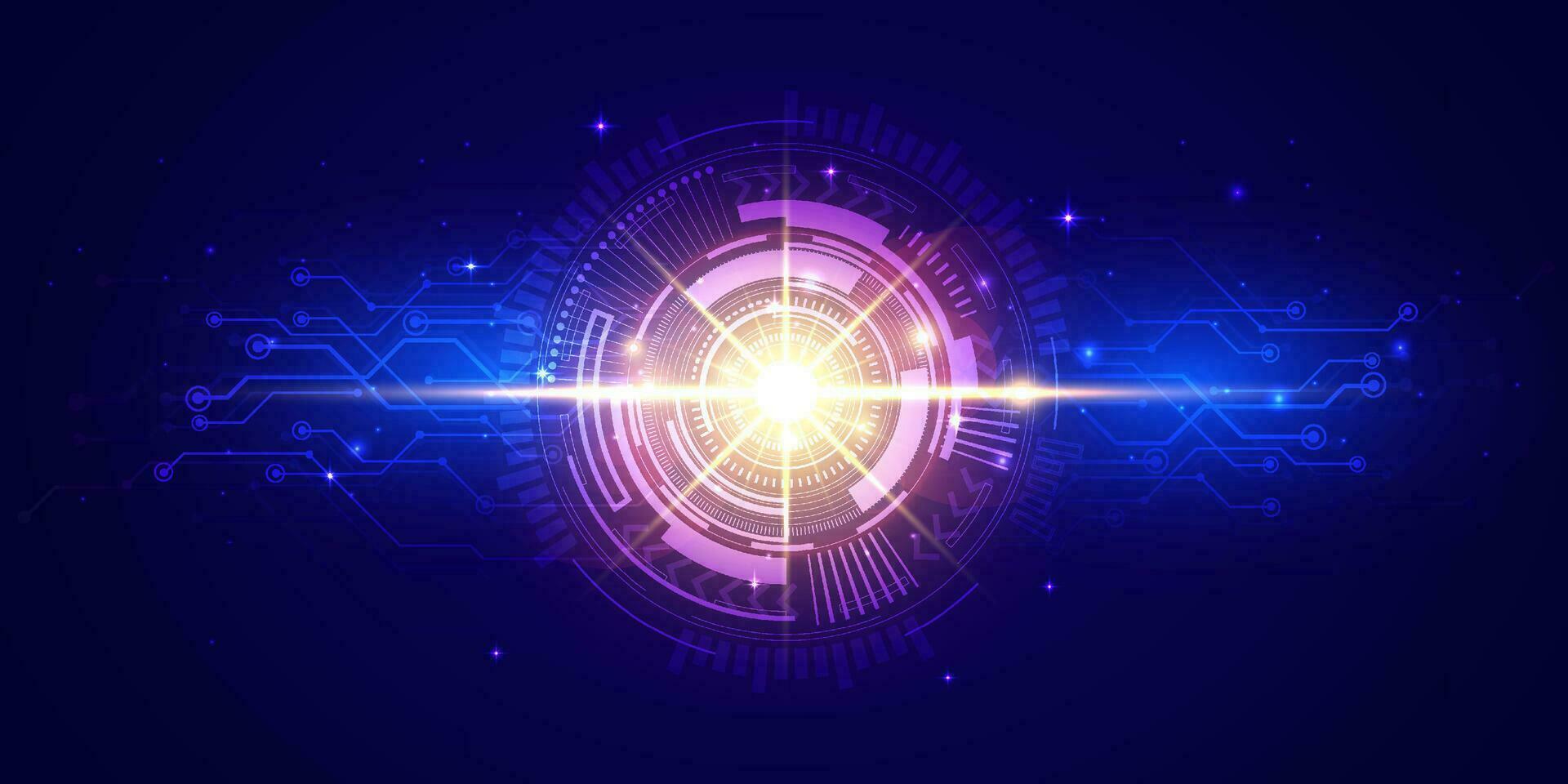The image is a digital painting featuring a science fiction-inspired abstract design. The background transitions from black in the four corners to light blue as it progresses inward. On both the left and right sides, light blue lines and dots create patterns reminiscent of circuit board pathways. At the center is a large, glowing yellow circle radiating beams of light, resembling a bright sun or star. Surrounding this central light source are intricate purple and pink concentric circles interconnected by various lines and shapes, much like the intricate networking of a circuit board. The overall composition is topped with interconnected blue squares and lines, creating a dynamic and futuristic visual. The dark blue background is speckled with light blue dots, reminiscent of stars in a night sky, enhancing the otherworldly feel of this vibrant digital artwork.